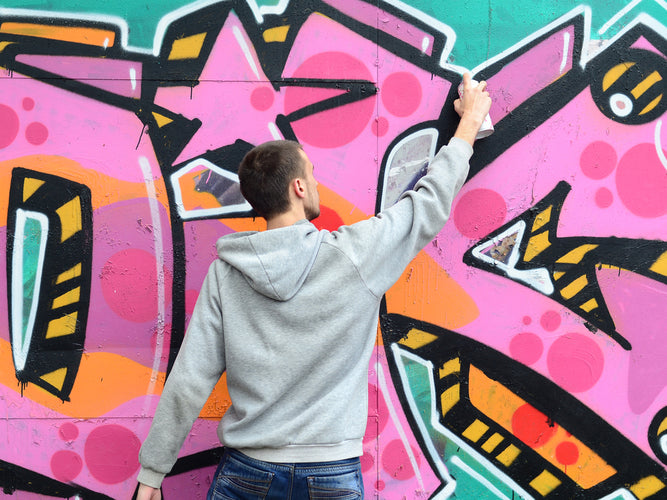The image captures a graffiti artist, a white male with closely cropped brown hair and a slight beard, in the process of creating a vibrant mural. He's seen from the back, wearing a gray hoodie and blue jeans, with his right arm raised, holding a white spray can, and his left hand partially visible. The mural itself is a dynamic composition of various colors and shapes, prominently featuring patterns in pink with deeper pink circular accents and a black outline. The top of the wall is painted green. 

On the right, there's an arrow with yellow and black stripes, and to the left, a rectangular shape with a similar pattern. The mural includes a mix of abstract and geometric forms, such as large reddish circles on a pink background, a thick black line forming a triangle, and a section resembling a field of oranges. There's also a black arc near the top, and elements like a five-pointed star with pink and red interior, surrounded by intricate black lines.

Other details include an orange shape with a black panther-like outline, white and sky blue elements, and an uneven turquoise shape. Smaller components like orange trapezoids, rectangles, and triangles are interspersed throughout. The entire piece suggests a rich, multifaceted design, blending a mix of motifs and colors against what appears to be a concrete wall.